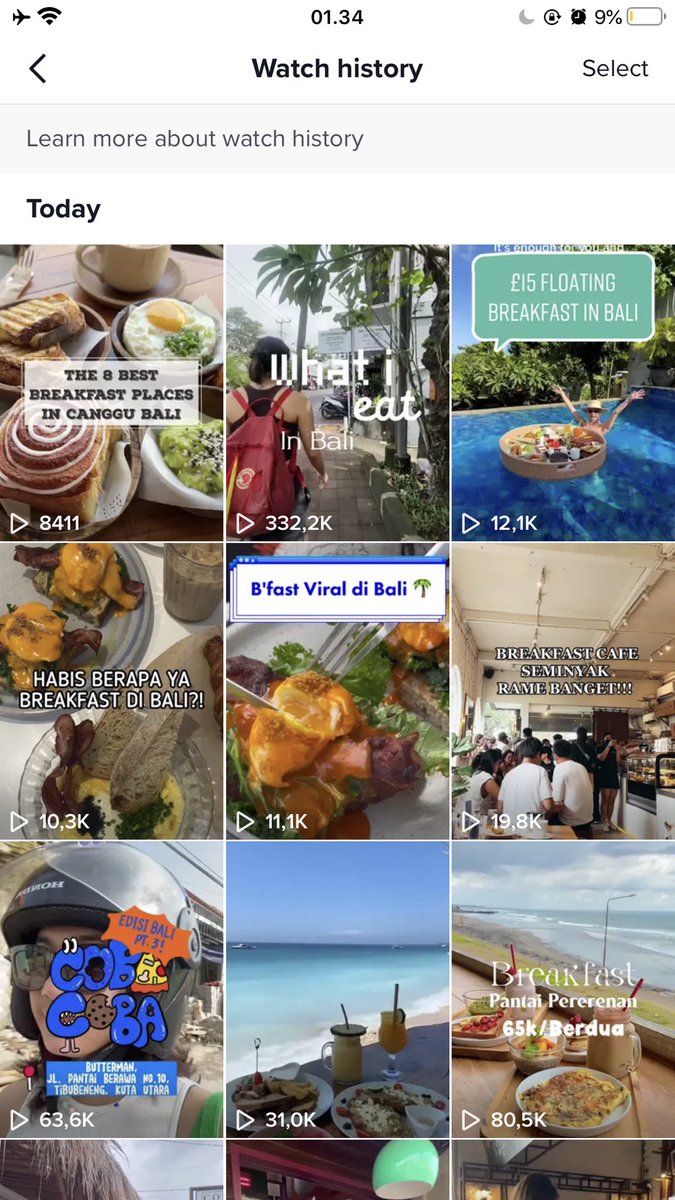**Detailed Caption:**

This screenshot captures the watch history of a social media platform, potentially TikTok or Pinterest, as viewed on a smartphone. At the very top of the screen, the phone status bar is visible, indicating the device is in airplane mode, connected to Wi-Fi, with a battery level of just 9%, and displaying the time "1:34".

Below the status bar, the interface prominently titles the page "Watch History", flanked by options such as "Select" on the right, and a link saying "Learn more about watch history".

Following this header, the main content reveals four rows, each containing three thumbnail images corresponding to recently watched content. The section is labeled “Today”.

- **First Row:**
  1. An image depicting food.
  2. A video titled "What to Eat: What I Eat in Bali".
  3. A thumbnail for "$15 Floating Breakfast in Bali".

- **Second Row:**
  1. A video titled "Habits", with the rest of the text written in a non-English script.
  2. Similar to the previous thumbnail, another video titled "Habits" with text in the same foreign language.
  3. An image titled "Breakfast Cafe Seminar Rami Banget", suggesting a popular seminar centered around breakfast cafes.

- **Third Row:**
  1. A stylized image with a cartoon overlaying a girl's face, captioned "Coba Coba".
  2. A scenic shot of food and drink set against a backdrop of the ocean.
  3. Another picturesque breakfast setup by the ocean.

This watch history details a user's eclectic culinary interests with a focus on meals, particularly breakfast, and scenic dining experiences, often related to Bali.